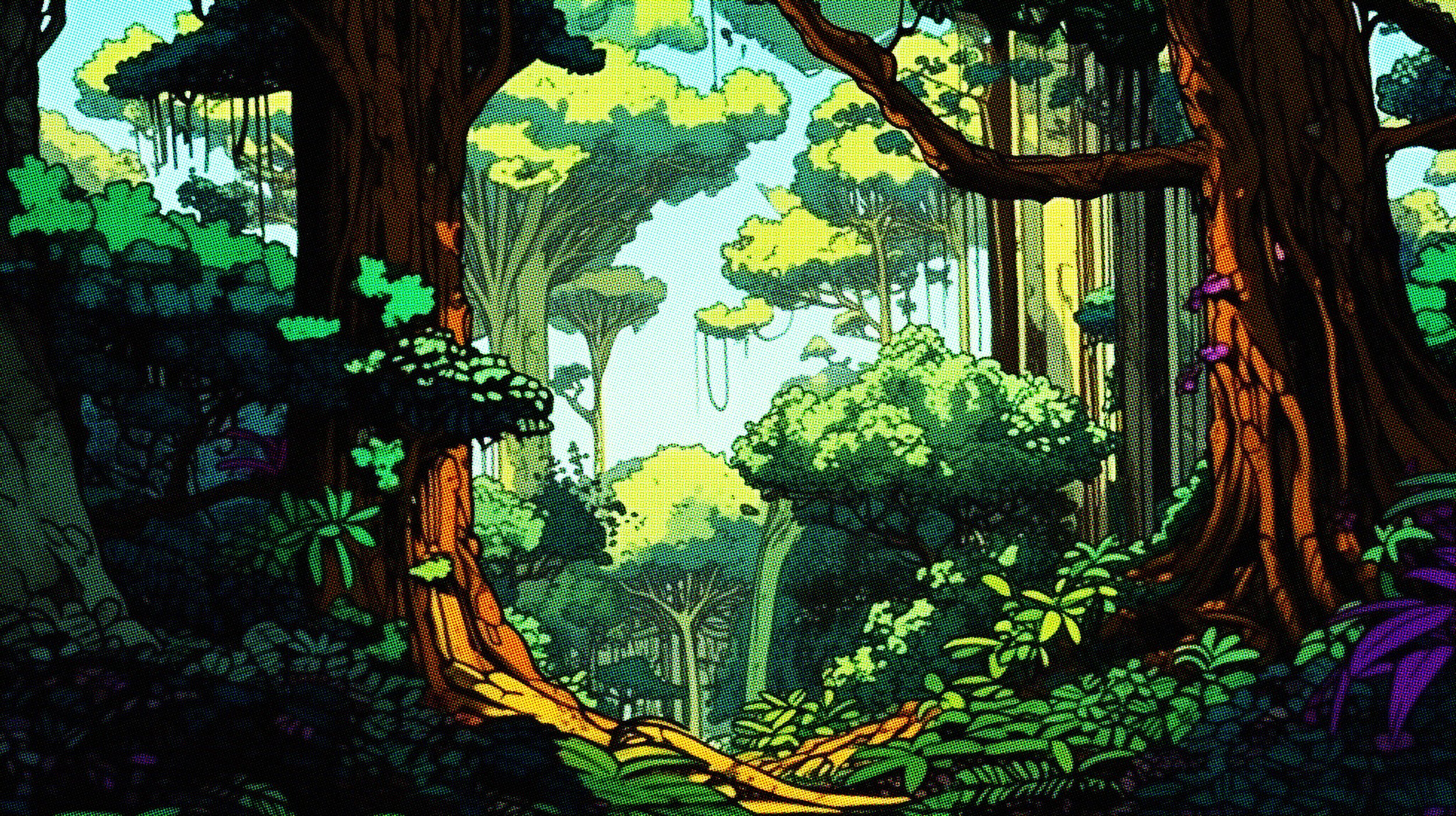The animated, cartoon-like image depicts a vibrant jungle or forest setting under a clear blue sky. Dominated by shades of green and brown, the scene is filled with numerous trees, some with tall trunks and leafy tops, while others have vines hanging like ropes. In the foreground, two prominent brown trees grab attention—one on the left with a canopy resembling a mushroom top, illuminated by sunlight at its roots, and another on the right with a branched extension that reaches into the center of the image, adorned with patches of purple fungus. The forest floor is covered in a rich layer of green plants, mixed with bushes, and a distinctive plant with purple leaves in the bottom right corner. The overall scene evokes the colorful, lively aesthetic of "The Land Before Time," blending various greens and browns with touches of purple. The background is a dense array of green trees, adding depth and richness to the forest environment.